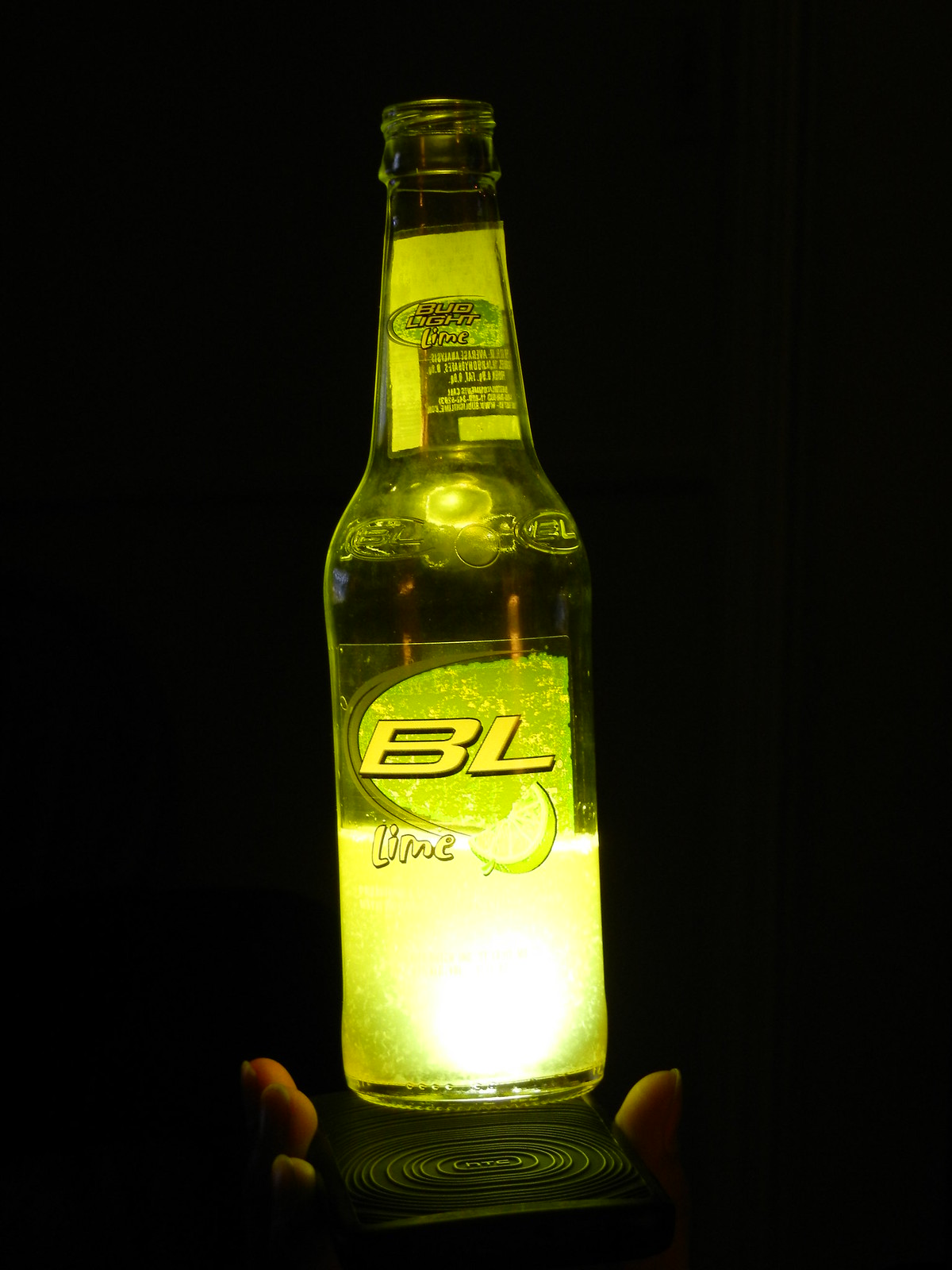In a striking image taken in a dark room with a black background, a clear glass bottle of Bud Light Lime is being illuminated from below by the flashlight of a cell phone, creating a captivating green glow that shines through the bottle. The label prominently displays "BL" in white letters, accompanied by an image of a lime wedge and the word "lime." At the top of the bottle, "Bud Light Lime" is inscribed again along with additional product information. The bottle is held by a hand with longer fingernails, adding a personal touch to the otherwise minimalist and neon-lit composition.